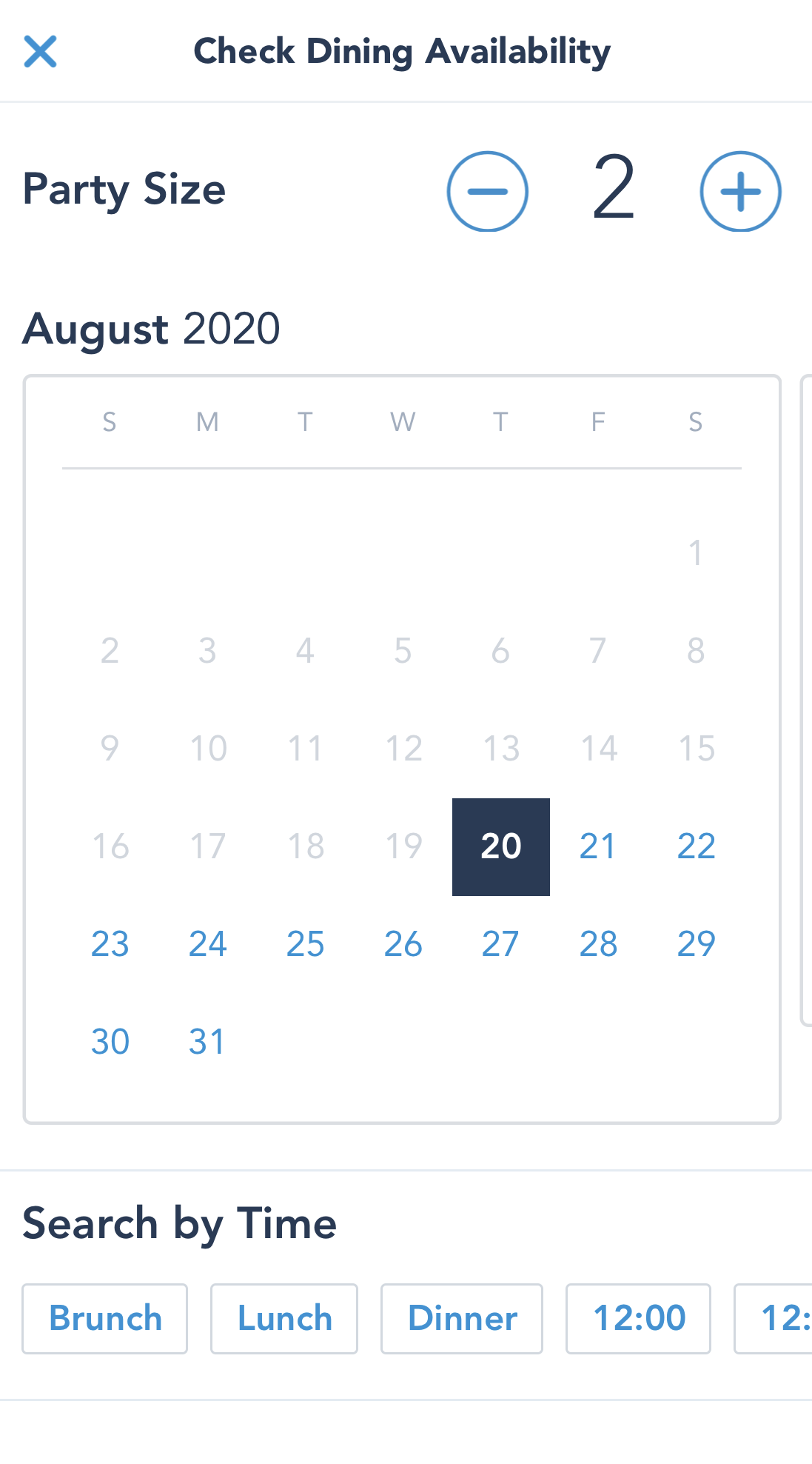This image showcases a user interface for checking dining availability on a predominantly white background, accented with blue, black, and grey text. At the top of the page, there is a header that reads "Check Dining Availability," accompanied by a blue "X" icon to close the window. 

Below the header, the "Party Size" section allows users to adjust the number of people in their party with a minus button, the number 2 displayed, and a plus button to increase the size. 

Further down, the "Date" section displays a calendar set to August 2020. The dates between August 1st and 19th are greyed out, while dates from August 20th to 31st are in blue. August 20th is specifically highlighted with a navy blue box and white text, indicating it is the selected date. 

The "Search by Time" section features buttons labeled "Brunch," "Lunch," and "Dinner," all styled with blue text on white boxes.

This image appears to be part of an application or webpage designed for users to check the availability of dining reservations. It illustrates the functionalities for adjusting party size, selecting a date, and searching by meal times.